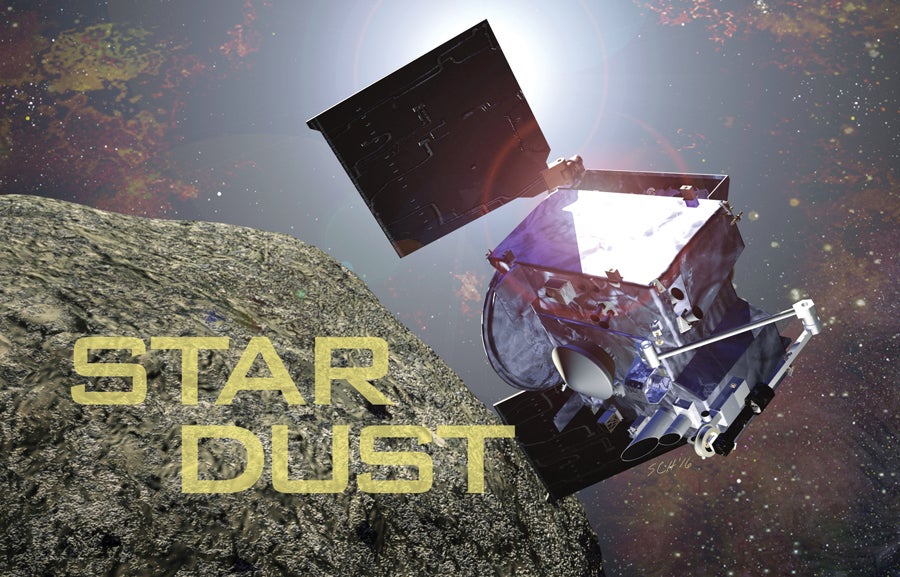In the image, a detailed scene in outer space is depicted. Dominating the bottom left is a large, mottled asteroid with a vein-like pattern, presenting a textured, gray, and slightly greenish-yellow surface akin to sandpaper. Written atop the asteroid in capitalized, blocky yellow font are the words "STARDUST," with "STAR" above "DUST," both prominently displayed. The background consists of a dark expanse speckled with red, yellow, and brown star-like formations, alongside cloudy star formations and subtle sun flares. To the right, a sleek satellite floats, composed of various reflective silver structures and black solar panels. The satellite appears mostly gray, white, and blue, and one of its components captures incoming light. Below the satellite, the letters "SCH16" can be discerned, indicating the author's mark. A prominent white beam of light illuminates the center of the image, adding to the cosmic ambiance.